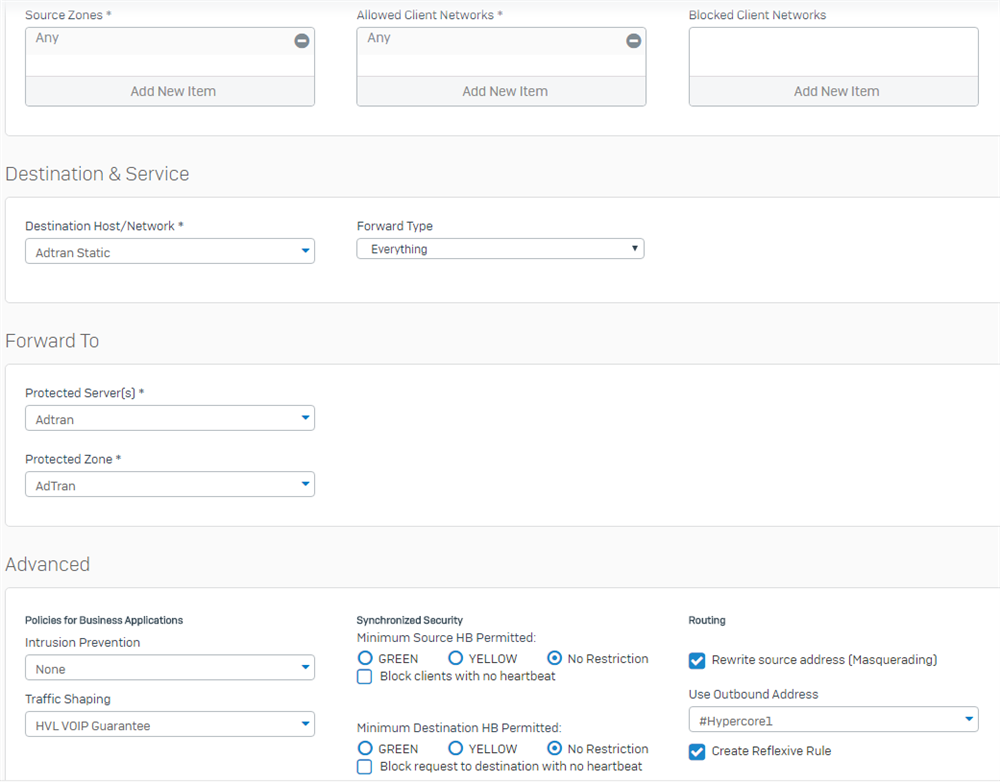This image depicts a detailed, multi-section form designed for database entry. The form is neatly divided into various segments, each with specific fields and options.

### Top Section:
- **Source Zones:** Contains a rectangle labeled with "Any," alongside a black circle with a line through it.
- **Allowed Client Networks:** Similarly, this section has a rectangle marked "Any," accompanied by a black circle with a line through it.
- **Blocked Client Networks:** Features a blank rectangle without any inscriptions.

### Divider:
- The form is bisected, with each section at the bottom containing a slightly gray area labeled "Add New Item."

### Middle Section:
- **Destination and Service:**
  - **Destination Host Network:** Star icon with a dropdown menu denoted by a blue downward arrow labeled "Add Trans Static."
  - **Forward Type:** Enumerable options under a blue downward arrow labeled "Everything."
  
- **Forward To:** 
  - **Protected Servers:** Dropdown menu labeled "Add Tran."
  - **Protected Zone:** Positioned below "Protected Servers," also featuring an "Add Tran" option with a downward arrow.

### Advanced Section:
- Various fields dedicated to:
  - **Policies for Business Applications**
  - **Intrusion Prevention:**
    - Dropdown menu set to "None"
  - **Traffic Shaping**
  - **HLV** 
  - **VoIP Guarantee:** Accompanied by a downward arrow.
  
- **Synchronized Security:** 
  - **Minimum Source HB Permitted:** Includes three circular options with "No Restriction" highlighted by a blue dot.
    - Additional circles labeled "Green" and "Yellow."

  - **Block Clients with No Heartbeat:** Represented in a square.

  - **Minimum Destination HB Permitted:** Reflects the same fields as the minimum source HB, with "No Restriction" selected.

### Right Section:
- **Routing:**
  - Checkbox highlighted in a blue square labeled "Rewrite Source Address."
  - Option labeled "Create Reflective Rule" with a checkbox.

This form is designed to facilitate comprehensive data entry, ensuring detailed specification and configuration across various network and security parameters.